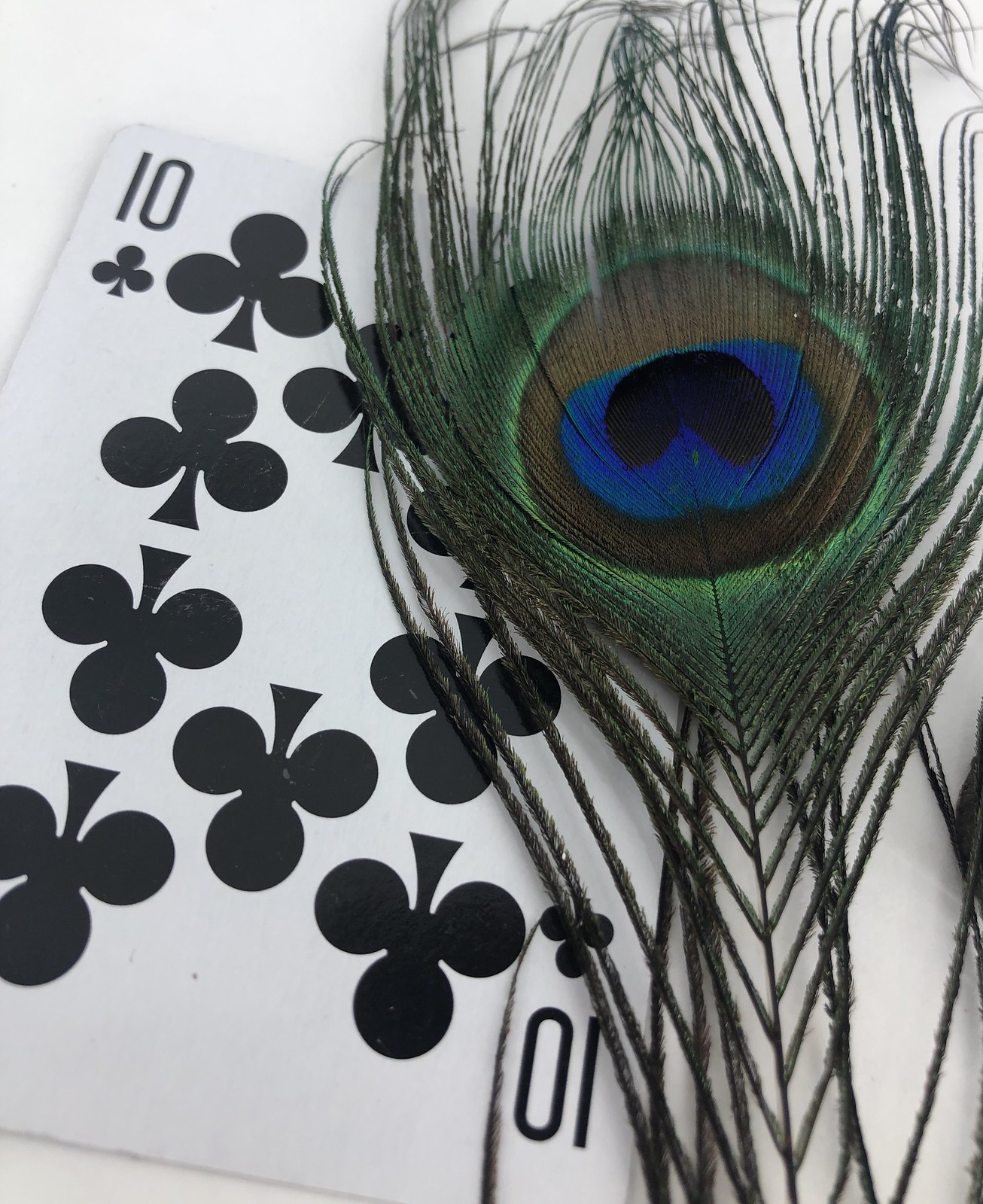This image features a single peacock feather resting atop a white playing card, specifically the Ten of Clubs. Though the lighting is dim, the feather's intricate beauty can still be appreciated. The lower part of the feather is a deep, velvety green, leading up to lighter green segments and culminating in the signature "eye" of the feather. This eye is composed of several distinct concentric layers: it begins with a pale green outer ring, followed by a dingy copper band, then transitions into a vivid, bluish-purple indigo, and finally centers around a black shape resembling an upside-down Pac-Man or a pie missing a slice. Despite the subdued light, the texture and detailed coloration of the peacock feather are fascinating, with each delicate strand contributing to its overall allure. The feather lies prominently on the right side of the card, drawing attention to its elegant form juxtaposed against the stark simplicity of the playing card beneath it.